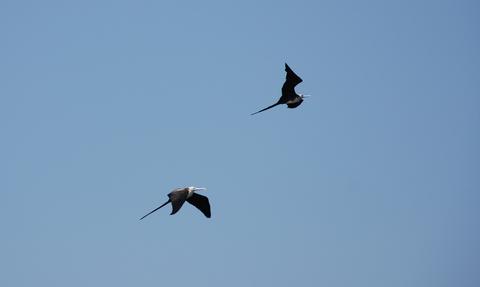In this blurry, low-resolution digital image, two large seabirds with distinctive features are captured flying against a clear, flat blue sky. The birds, possibly pelicans judging by their large beaks and significant wingspans, have black wings and white heads. The bird at the top of the image is seen with wings upward in mid-flap, while the one at the bottom has its wings pointing downward. Both birds are soaring upward from the bottom left towards the top right quadrant of the image, their slender tails trailing behind them. Despite the poor quality of the photograph, the general outline of the birds remains discernible, though finer details are muddled, making it challenging to precisely identify the species.